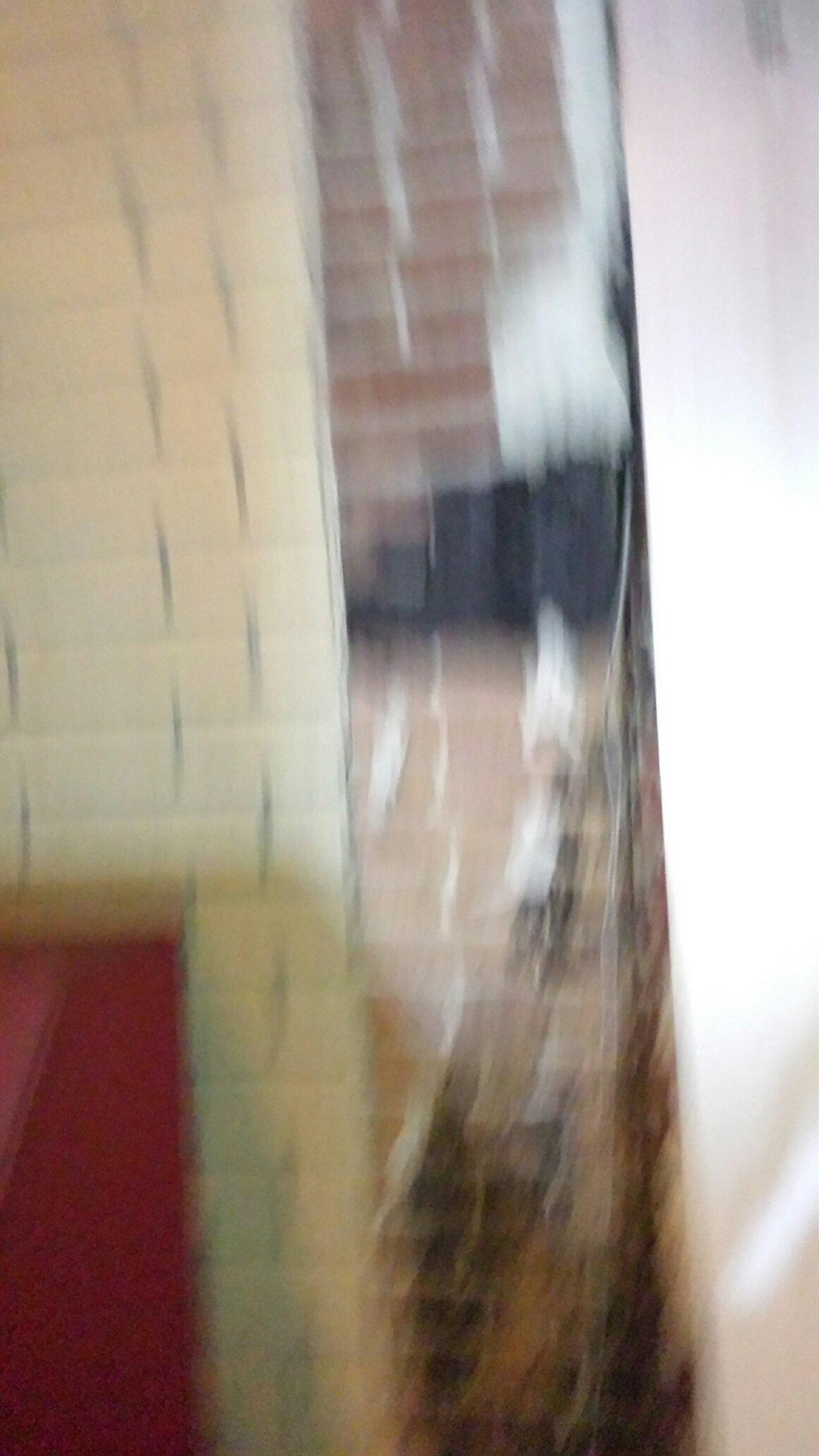This photograph, though blurred and elongated vertically, showcases a detailed brick wall as its primary focus. Dominating the center of the image, we observe traditional red-colored bricks forming part of what appears to be a small mantel or shelf. As our eyes move to the left, the brick pattern transitions, displaying lighter-colored bricks that contrast the rest of the wall. This lighter section leads down to the lower left corner, revealing the hearth of a shallow fireplace adorned with a red background. This fireplace seems to be a supplementary addition beside a chimney, which occupies the central portion of the image. The right side of the photograph features a stark white wall, providing a clear distinction from the intricate brickwork on the left. The angled brick design further supports the interpretation of the left side as the upper and lower segments of the fireplace, rather than a doorway.